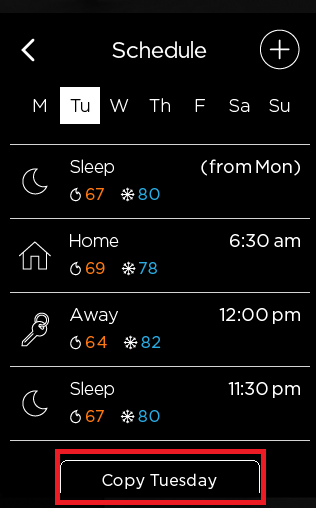The image is a cell phone screen capture displaying a detailed schedule interface on a rectangular black background. At the top center, there is a white arrow pointing to the left. Subsequent to the arrow, the word "Schedule" is written, with a capital 'S'. To the right of "Schedule," a white circle containing a cross is visible.

Beneath this heading, the days of the week are listed using their initial letters: M, T, W, Th, F, Sa, Su, all in white. Tuesday (Tu) is highlighted with a white square around it. Below the day indicators, a horizontal white line segments the next section.

The next section begins with a white-bordered crescent moon icon, followed by the word "SLEEP" in capital letters. Below this is a white-bordered icon resembling a droplet or possibly a temperature marker, with the number "67" in orange text next to it, indicative of a temperature. Adjacent is a blue "80" with a snowflake icon, denoting the temperature range.

To the right, within parentheses, it reads "Mon" (with the 'M' capitalized) and is capped off by another white line stretching horizontally. Below, there is a white-bordered drawing of a house front with the word "Home" capitalized next to it. The following details are displayed: an orange "69" with a small flame icon and a blue "78" with a snowflake icon. The time "6:30 AM" is situated in the upper right corner.

Further down, another icon appears on the left resembling a key with a key ring, signifying "Away" in capital letters. Below this, the temperatures "64" in orange and "82" in blue are displayed with respective indicator icons. The time "12:00 PM" is noted at the right-hand corner.

A subsequent section features another white line, a crescent moon icon with the word "SLEEP" in capital letters to the right, and detailed temperatures: "67" in orange with a flame icon and "80" in blue with a snowflake icon. The time "11:30 PM" is indicated here.

Finally, at the bottom, a red-bordered rectangle with vertical white lines inside it (left and right) is present. Below this, the words "Copy Tuesday" are written, with the "C" and "T" capitalized.

This image illustrates a detailed and structured schedule interface, highlighting different temperature settings for home, sleep, and away modes, along with timestamps and symbolic icons for ease of use.